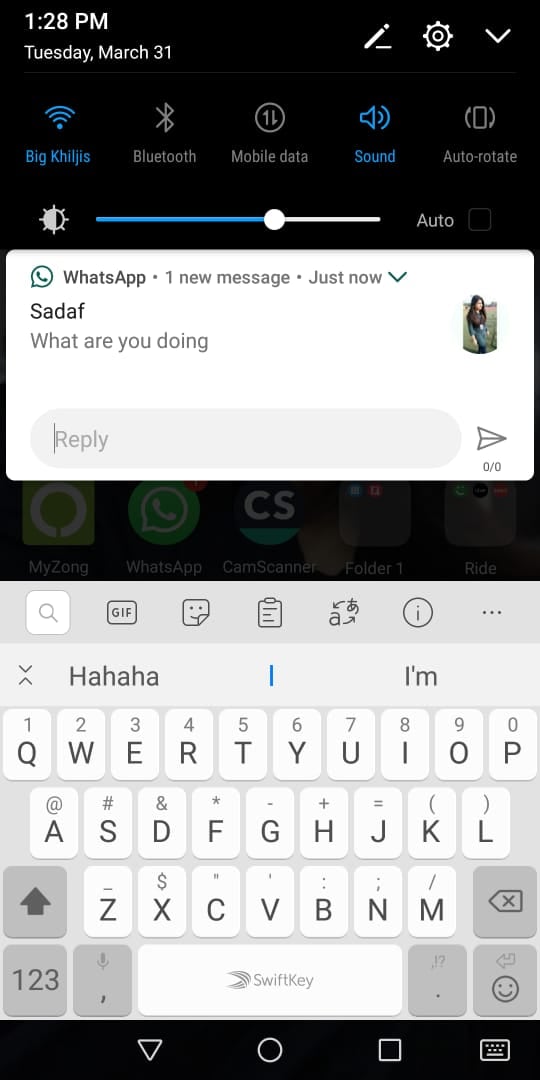A detailed description of the screenshot includes:

The screenshot displays a smartphone screen at 1:28 PM, visible on the top left corner. The device is in dark mode, featuring a black background. The notification bar is open, showing a connected wifi network named "Big Kijis" highlighted in blue. Other icons visible in the notification bar include Bluetooth, mobile data, sound, and auto-rotate. Below this, a brightness adjustment slider is present.

A WhatsApp notification is visible, indicating a new message from a contact named Sajaf, asking, "What are you doing?" with an option to reply. Sajaf's profile picture is displayed to the right of the message. The virtual keyboard occupies the bottom part of the screen. In the background, between the WhatsApp notification and the keyboard, several app icons are partially visible: MyZong, WhatsApp, CamScanner, FoldTea, and Ride.